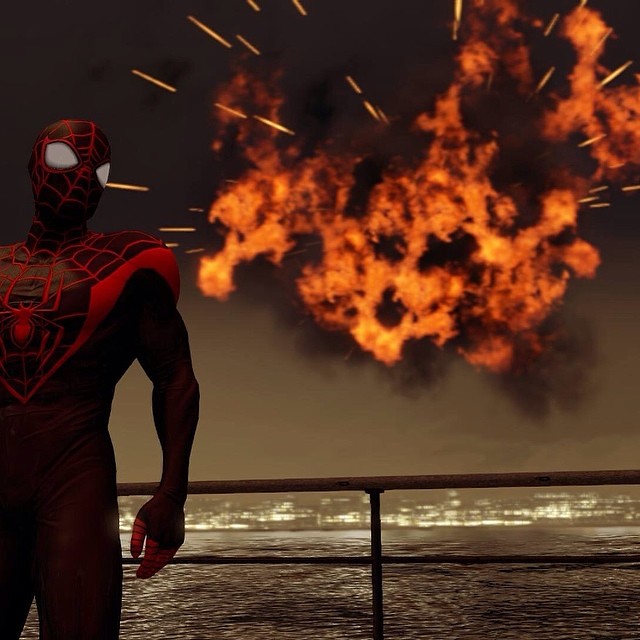In the image, Spider-Man is prominently featured on the left-hand side, with approximately three-fourths of his figure visible. He is garbed in a dark blue Spider-Man suit adorned with the iconic red spider web pattern that spans from his chest up to his head. His mask features large, white eye openings that are characteristic of the superhero. In the background, a dramatic explosion engulfs the scene with vivid orange flames, casting an intense glow. A railing separates Spider-Man from the chaotic backdrop. Beyond the explosion, a body of water reflects the surrounding elements, leading the eye toward a brightly lit cityscape in the distance, characterized by numerous twinkling white lights. The overall composition presents a stark contrast between the calm city and the fiery turmoil in the foreground.